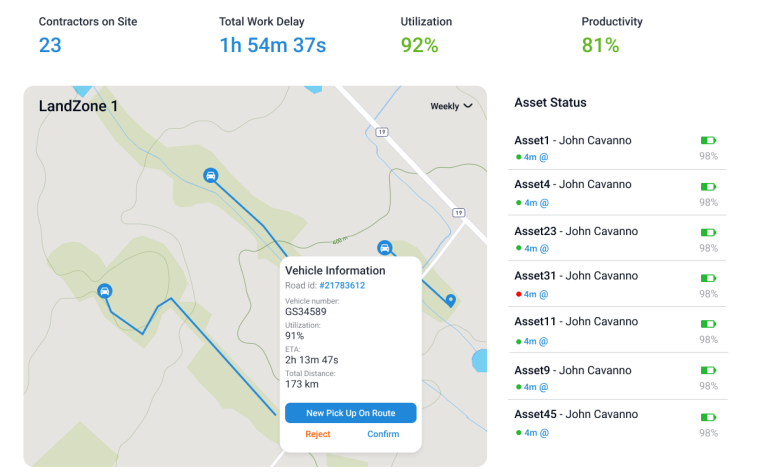This image showcases a screenshot of a detailed map interface used likely for project management or logistics. At the top, four informative columns in black text provide key metrics: "Contractors on Site: 23," "Total Work Delay: 1 hour, 54 minutes, 37 seconds" (in blue text), "Utilization: 92%" (in green text), and "Productivity: 81%" (also in green text). Below these columns, the layout splits into a map on the left and a sidebar on the right.

The map prominently features labels "Land Zone 1" in the top-left corner and "Weekly" in the top-right corner. In the lower right area of the map, a white overlay window presents "Vehicle Information." Within this window, "Road ID Number 21783612" appears in blue at the top, while at the bottom, there is a blue button labeled "New Pickup on the Route." Beneath this button are two options: a "Reject" button on the left and a "Confirm" button on the right.